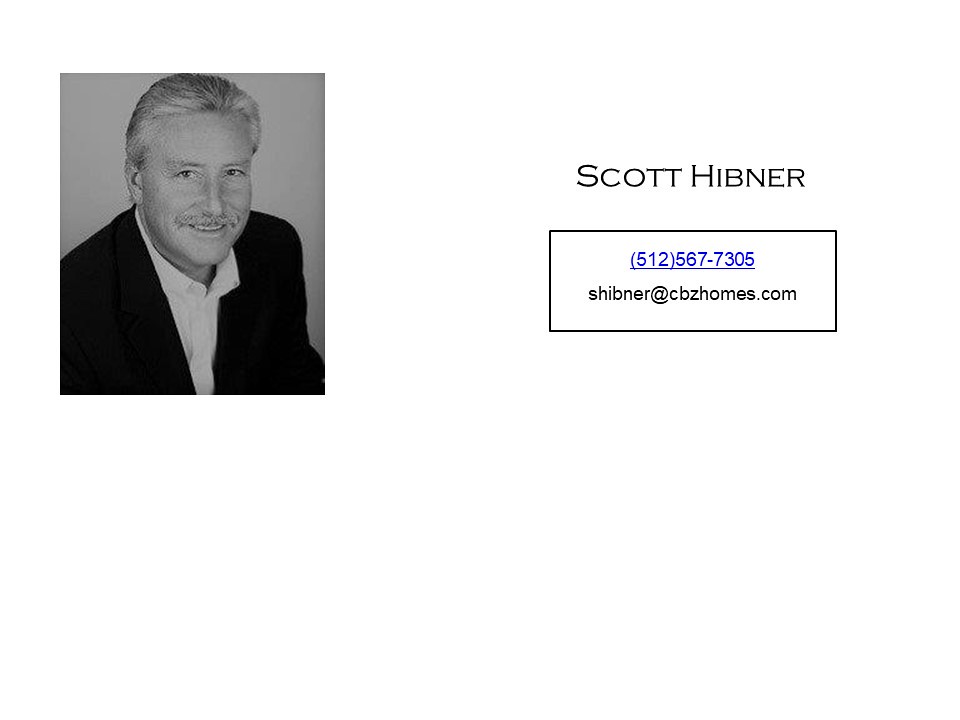The black and white image features a headshot and torso of a man named Scott Hibner, dressed in a white button-up shirt with a collar and a black jacket. He has whitish-gray hair and is smiling at the camera. The background of the image is gray. Positioned to the right of his photo, there is black text on a white background displaying his name, "Scott Hibner," with the spelling "S-C-O-T-T H-I-B-N-E-R." Directly below his name is his phone number, "512-567-7305," in blue text. Beneath the phone number, it reads "S.Hibner at CBZHomes.com." The overall layout and design suggest that the image may be part of a business card or a professional flyer, with Scott's image to the left and his contact information neatly organized to the right, positioned next to his face for easy readability.